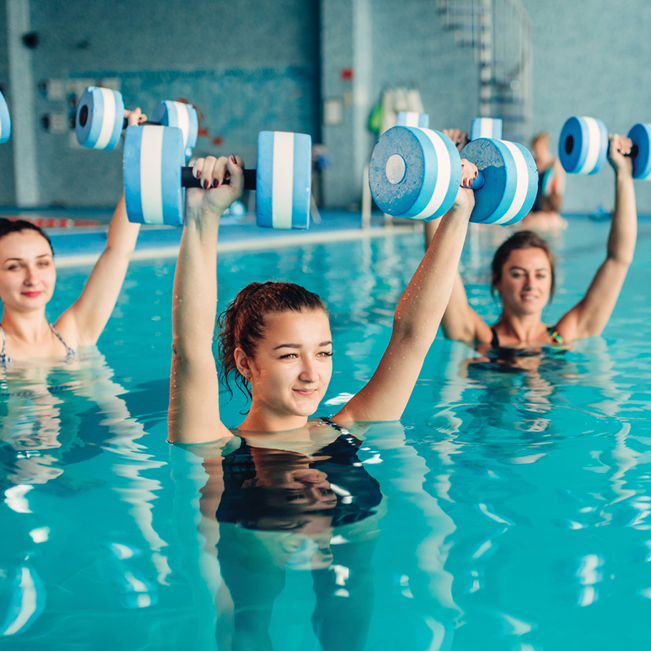In this realistic, square-shaped photograph of a large public pool, three young women are engaged in an aqua fitness class. Positioned front and center, the women, who are white and have black hair, are clad in swimsuits, and each lifts a pair of styrofoam dumbbells with blue and white floatation discs and black handles above their heads. They all smile warmly, looking towards the camera. The pool’s clear blue water reaches up to their shoulders, emphasizing the immersion in their workout. Behind them, there's minimal activity, with one or two blurry figures seated at the pool's edge. The background features a blue-tiled wall adorned with signs and a distinctive blue and white spiral staircase that intriguingly rises from the rear of the pool area. The overall atmosphere is bright and inviting, capturing the essence of a well-kept aquatic facility and the enthusiasm of the participants.